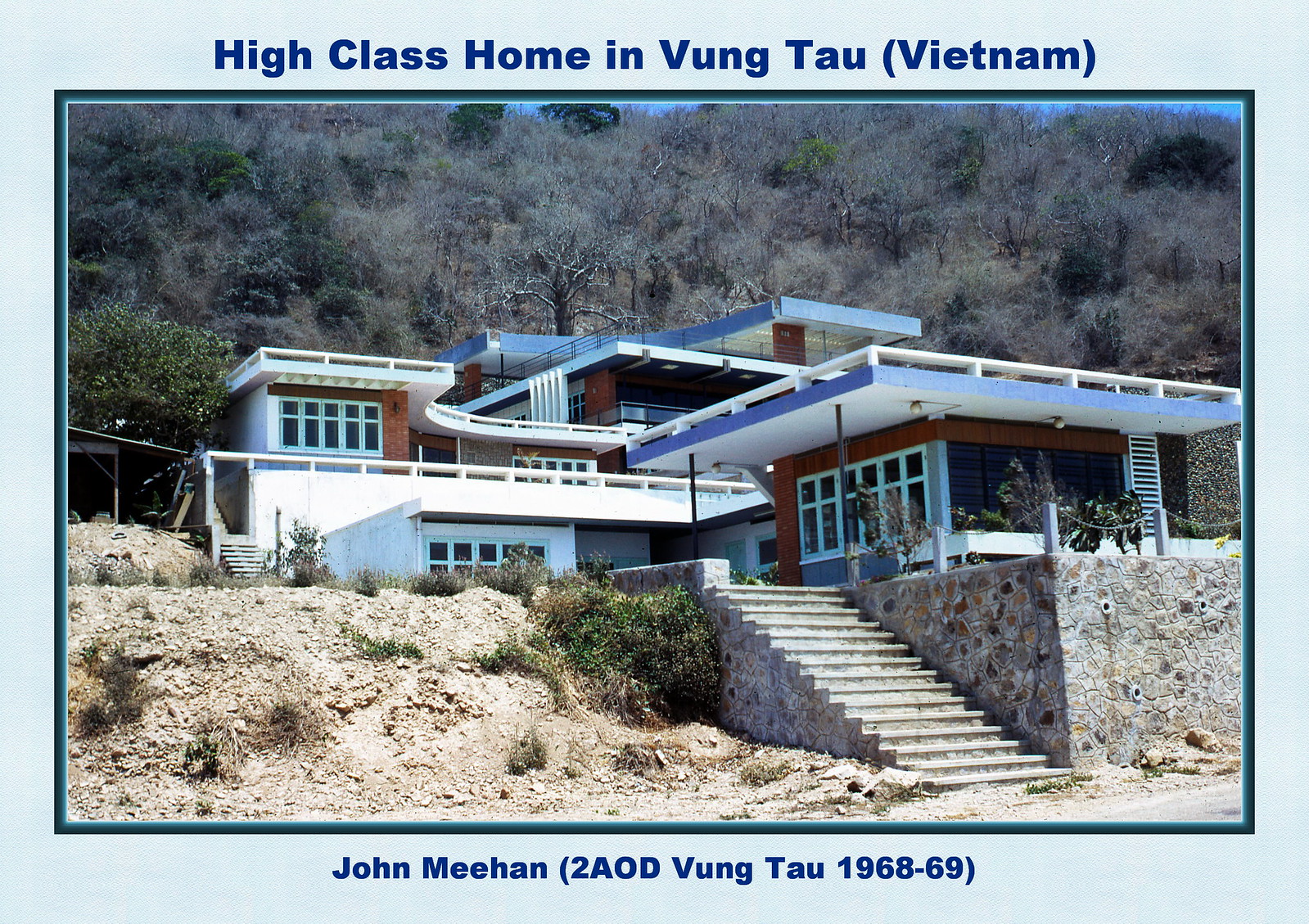This is a meticulously detailed postcard featuring a grandiose house located in Vung Tau, Vietnam, dated from 1968 to 1969. The house, resembling a celebrity mansion, is an imposing four-story structure with a distinctive square design and extensive stone walls. The construction evokes the style of high-class homes seen in Los Angeles, connoting luxury and exclusivity. The residence is set atop a hill, surrounded by dirt piles and rocks, adding to its unique positioning. Greenery and bushes are scattered around, enhancing the natural beauty of the setting. The image is bordered by a blue frame, complementing the clear blue skies above. Inscriptions at the bottom of the postcard read, "Joe meet John Meehan," "High-class Homing Vung Tau, Vietnam," and "John Meehan to a OD Vung Tau 1968 to 69," in a dark blue text. The postcard captures a snapshot of opulence and intriguing architecture from the late 1960s Vietnam.